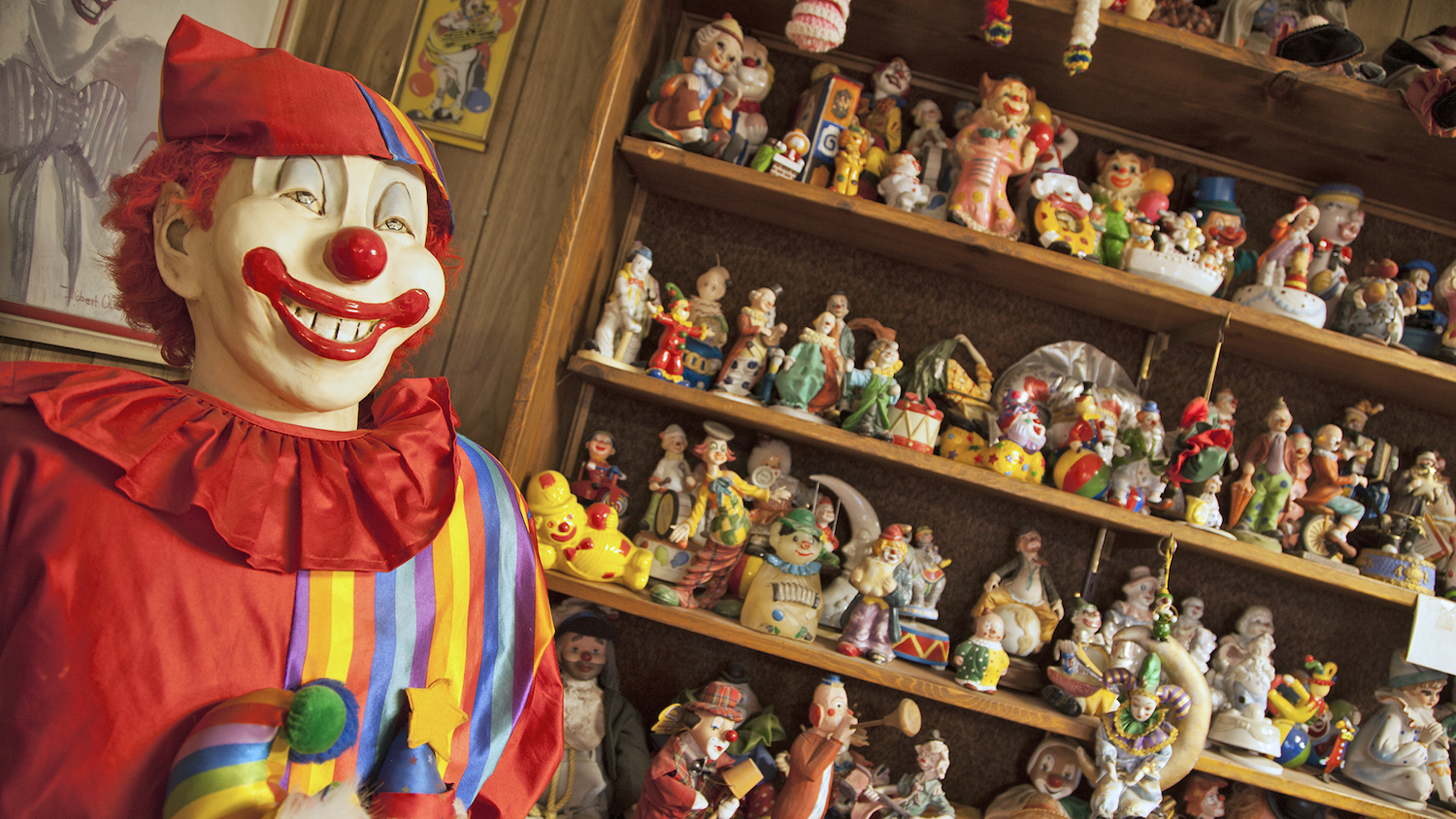The photograph captures the interior of a shop, specifically showcasing a richly detailed and eclectic collection of figurines predominantly themed around clowns. On the left side of the image stands a large, striking clown figure, visible from the chest up. The clown is attired in a vibrant red fabric hat adorned with rainbow stripes on one side, and it sports a white-painted face complete with a large red button nose, a wide red smile, and striking red hair. The clown's outfit features a ruffled red satin top with rainbow lines, adding to its flamboyant appearance.

Dominating the right side of the image is a wooden shelf, brown in color, affixed to a similarly wooden and brown-colored wall. This shelf comprises five levels, each crowded with a multitude of small figurines. The majority of these figurines are also clowned-themed, displayed in a variety of poses—some are perched atop bowls, while others are depicted playing musical instruments. These clowns come in various colors and styles, lending a lively and whimsical atmosphere to the scene. The photograph itself is slightly tilted to the right, adding an additional layer of eccentricity to the already quirky and vivid shop display.